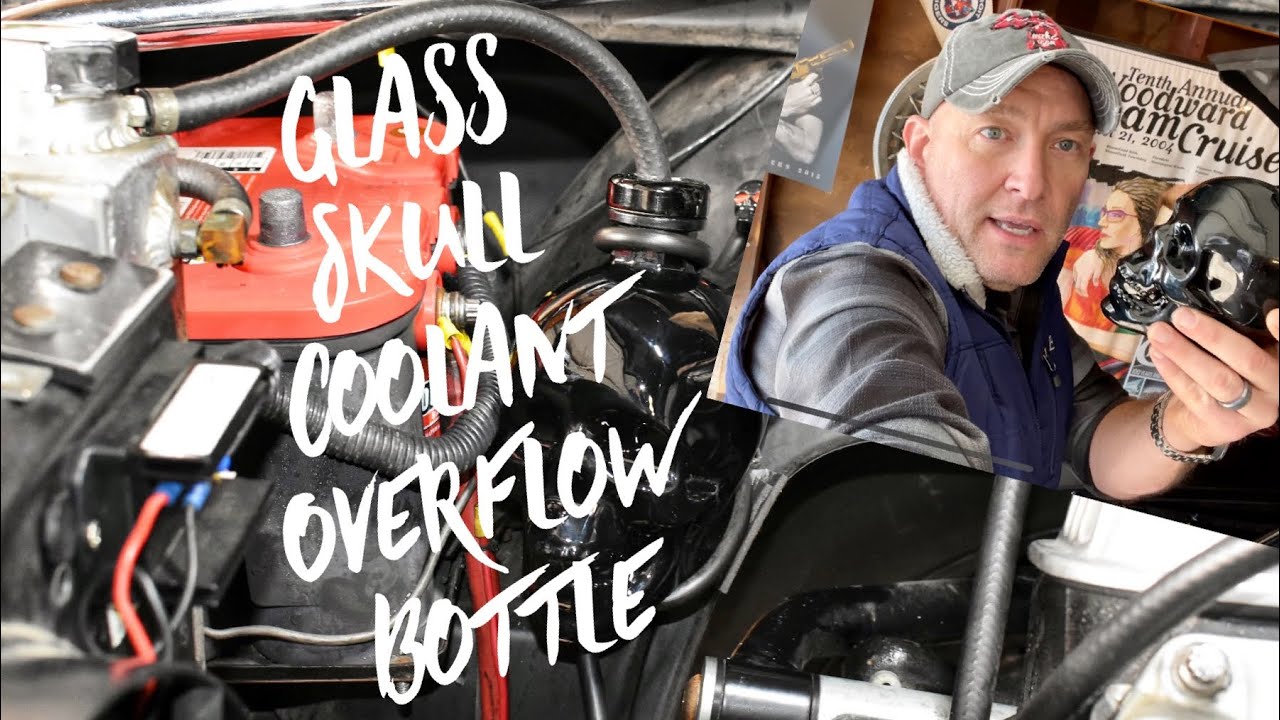The image is a horizontally oriented collage primarily showcasing parts of a car engine, including black and red components and some wires. Superimposed on the left side of the engine is white text in a loose handwriting style that reads "glass skull coolant overflow bottle." An opaque black glass skull is connected to the engine via a gray hose, indicating its function as a coolant overflow bottle. Overlaying the upper right portion of the image at an angle is a photograph of a middle-aged white man wearing a gray baseball cap with the outline of Michigan on it, a blue vest over a gray long-sleeve shirt, a silver wedding band, and a wristwatch. The man is holding the black glass skull up by his face and stands in front of a vintage poster that reads "10th Annual Woodward Dream Cruise 2004." The background features an image of a woman with brown hair in an orangish shirt, adding an additional layer to the collaged composition.